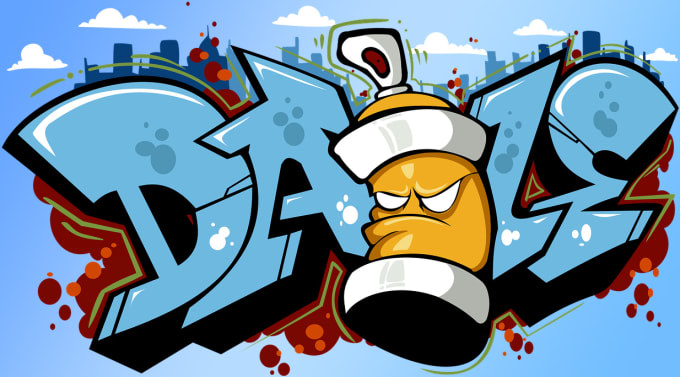The image showcases a vibrant, digital graffiti artwork featuring the word "DAZE" prominently in a dynamic graffiti style font. The letters are rendered in light blue with dark blue and white spots scattered across them, giving the text a textured look. Emanating from behind the letters are red splatter effects, adding depth and contrast to the design. In the center, between the letters "A" and "Z", is a cartoonish depiction of an anthropomorphized spray paint can, resembling an evil version of Bart Simpson with a yellow-orange face, and an angry, frowning expression. The character has stark white, pupil-less eyes and is topped with a large white spray nozzle. Below, the spray can features a black and white neckline. The backdrop of the artwork includes a cityscape silhouette shaded in various hues of blue, with a blue sky dotted with patchy white clouds. The sky surrounding the spray can character is lighter blue, adding a subtle highlight behind the central figure.